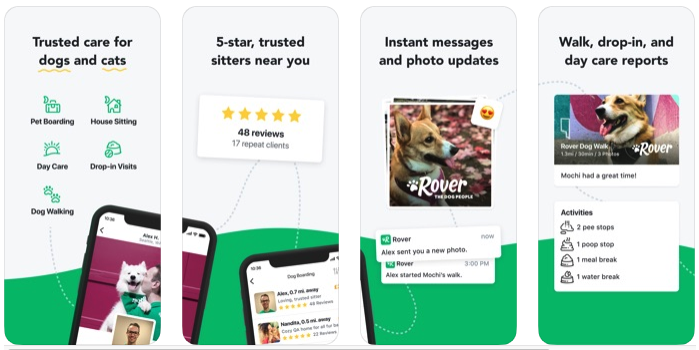Caption for the Rover promotional image:

The image features a collage of four square panels designed for Rover, a pet care service website. Each panel has a white top and green bottom section, with various pieces of informational text and images related to pet care services.

1. The first panel emphasizes "Trusted Care for Dogs and Cats," with the words "dogs" and "cats" highlighted in yellow. It lists various services such as pet boarding, house sitting, daycare, drop-in visits, and dog walking, each represented by a green icon. The image includes a cell phone showing a man kissing a large white dog as well as a separate picture of a Caucasian man wearing glasses.

2. The second panel highlights "Five Star Trusted Sitters Near You" and features five gold stars, followed by the text "48 reviews, 17 repeat clients." It depicts a cell phone with review information, including photos of a man and a woman, both providing five-star ratings.

3. The third panel showcases "Instant Messages and Phone Updates," featuring a brown and white dog and the Rover logo (R-O-V-E-R) with a paw icon. It displays a message notification from "Alex" with a photo update, indicating interaction through the Rover app.

4. The fourth panel outlines "Walk, Drop-In, and Daycare Reports" with the Rover logo and another image of the brown and white dog. It lists detailed activity updates, including "2 pee stops, 1 poop stop, 1 meal break, and 1 water break," each accompanied by corresponding icons.

This detailed collage underlines the comprehensive, trusted, and interactive services provided by Rover for pet care needs.